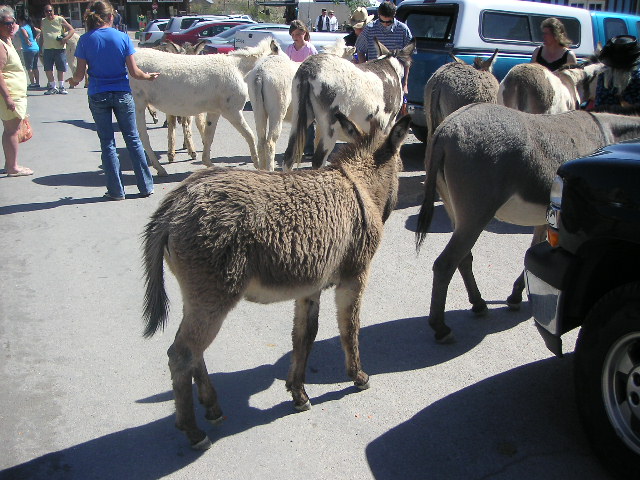This brightly lit daytime photograph captures a lively scene in a parking lot where numerous people and animals interact. In the background, several wooden buildings with screen doors are visible, alongside a variety of parked cars, including a white car, white SUV, red car, and a white pickup truck. A man and a woman, both wearing white shirts (the man additionally in a black vest), stand near the buildings. A person in a blue shirt and another woman dressed in yellow summer clothing are also notable among the group. At the forefront, a woman dressed in blue jeans and a blue shirt is seen petting one of the donkeys amongst seven to nine donkeys that roam freely. These donkeys come in various colors—grey, white, black, and brown, with one particularly recognizable by its black and brown markings. Additionally, a man in a blue striped shirt, near a blue pickup truck, appears to be feeding a donkey. This bustling scene suggests a park-like or fairground atmosphere during a sunny day.